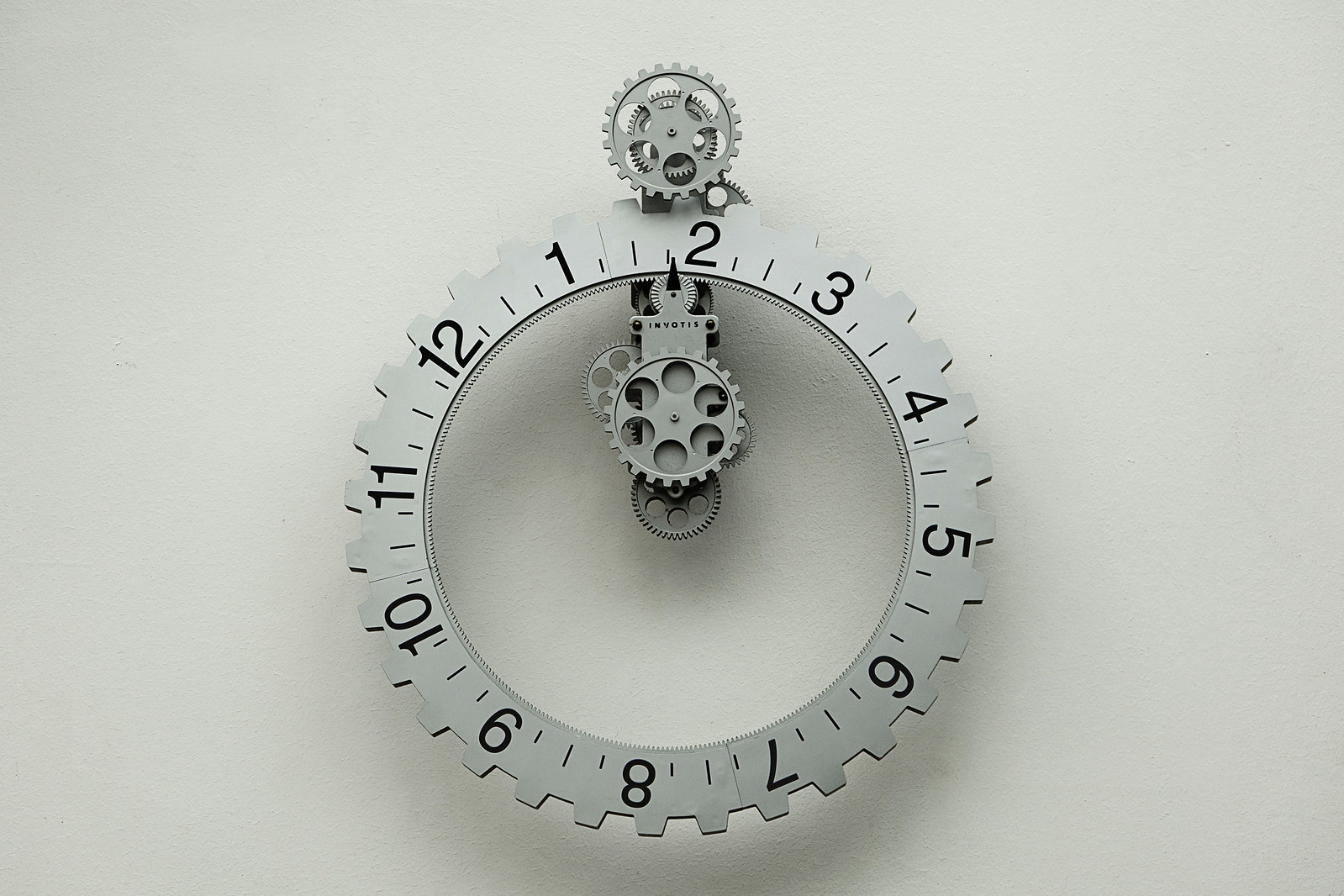This image depicts a silver, circular gear resembling the outer edge of a clock. The clock features black numbers from 1 to 12, arranged around the circumference, with the 12 offset to the top left, making it appear slightly turned sideways. The gear has teeth on its inner edge and houses additional gears at its center, which likely facilitate the movement of the outer gear. Towards the top, there are more gears that interact with the numbered dial, giving it a functional yet industrial appearance. The entire clock has a monochromatic grayish-silver tone, save for the black numbers and small hatch marks between them. The brand name "INVOTIS" is inscribed on one of the cogs. The clock, with its steampunk-inspired but minimalist design, is set against a stark white background, enhancing its mechanical details.